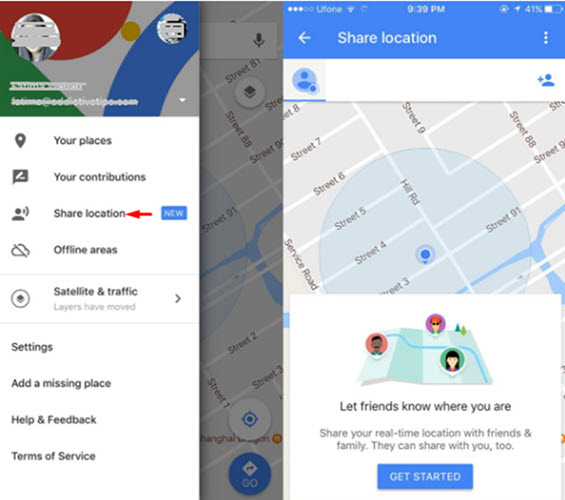This image is a screenshot capturing a Google Maps interface on a mobile phone. In the center, a semi-transparent overlay of two pop-up windows gives the display a blurred, hazy appearance. The prominent element in the middle is a map, showcasing a blue area likely representing water, surrounded by the predominantly white layout of streets, demarcated by white lines.

The left of the screen features a colorful vertical border. This border consists of a red section at the top left corner, green at the bottom left, and a horizontal white band in the center, which contains a yellow circle. The border transitions into blue stretching diagonally from the bottom left to the top right, and ends with a gray section in the bottom right corner. Two blurred profile pictures are positioned on the left and right sides of this vertical strip.

Beneath this border, there is a white menu with black text and corresponding icons. The first icon is a location marker labeled "Your places." This is followed by "Your contributions," and "Share location," which has a red arrow pointing to it on the right side and a blue tab labeled "New." Other options listed are "Offline areas," "Satellite and traffic," "Settings," "Add a missing place," "Help and feedback," and "Terms and service," all in a straightforward list format.

On the right side of the screen, a blue bar at the top displays the phone's status indicators: Wi-Fi, battery, and time. Beneath this status bar is a navigation section with a white left-arrow icon, the text "Share location" centered, and a vertical ellipsis (three dots) for a menu on the right. Below, another white bar holds the profile icons on both the left and right sides.

Further down, there's another map view, showing a street layout with a half blue circle emerging from the bottom and dark blue detailing within, set against light gray terrain and white streets. Below this map, a section prompts the user with text "Let friends know where you are," followed by additional lines of informational content and a prominent blue "Get started" button on a white background.